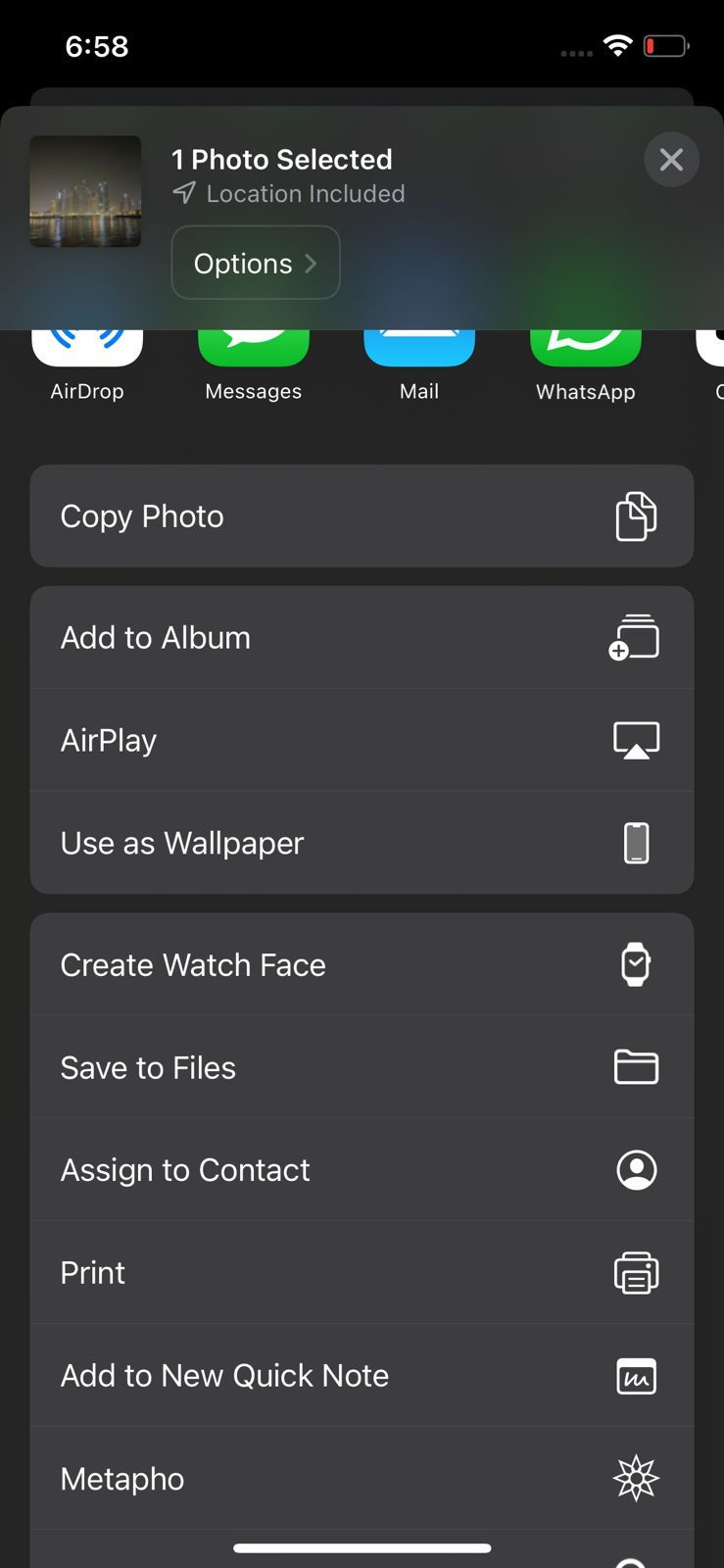This screenshot captures a person's cell phone interface. In the top left corner, the time is displayed as 6:58. The top right corner shows the Wi-Fi icon followed by a battery icon with a red bar, indicating the battery level is critically low. Below this, there is a captivating photograph of a city skyline at night. The bright lights of the skyscrapers reflect beautifully in the body of water in the foreground, creating a mesmerizing scene. 

On this screen, a banner reads "One photo selected," indicating that the image is selected and includes location data. Below this, various sharing and action options are listed: AirDrop, Messages, Mail, WhatsApp, Copy Photo, Add to Album, AirPlay, Use as Wallpaper, Create Watch Face, Save to Files, Assign to Contact, Print, Add to New Quick Note, and UFO.

The overall image has a portrait orientation (taller than it is wide), with a black background and white text. There are no people, animals, birds, plants, flowers, trees, automobiles, bicycles, or airplanes in this image.